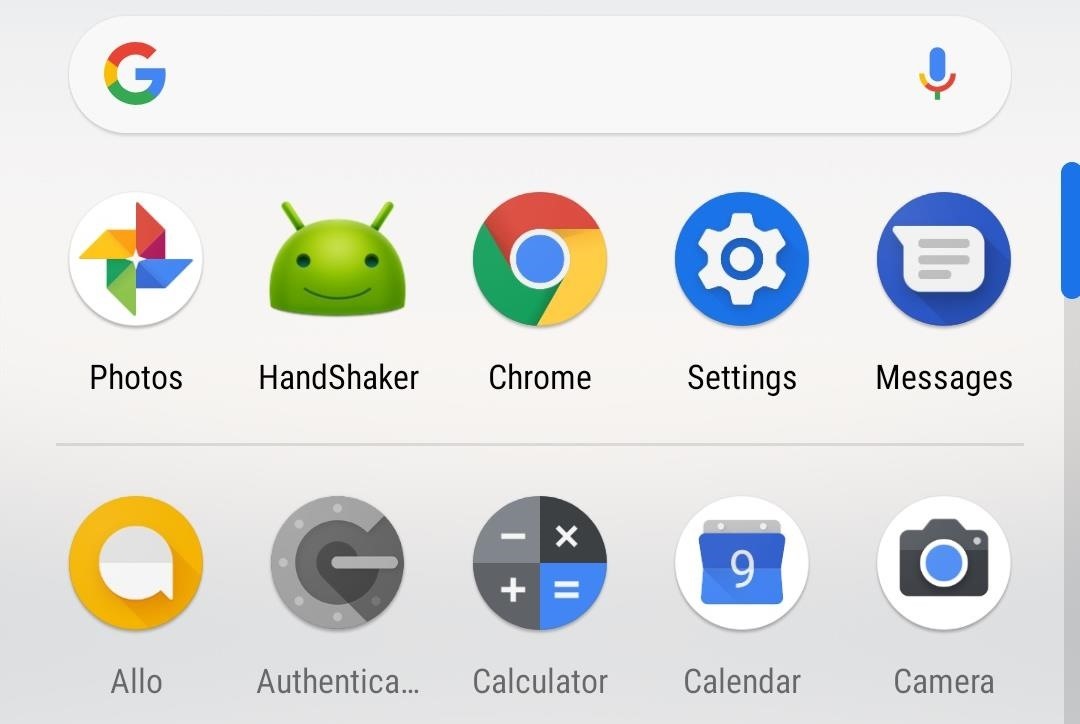The image depicts a section of a Google search interface on a mobile phone. The background is light gray, highlighting a search bar at the top of the screen. The search bar features the Google 'G' logo on the left side and a microphone icon in Google colors on the right.

Below the search bar, there are two rows of application icons. The first row includes:

1. Google Photos - represented by the Google Pinwheel icon.
2. Handshaker - featuring a green alien icon.
3. Google Chrome - depicted as a circle with Google colors.
4. Settings - shown as a white cog inside a blue circle.
5. Messages - indicated by a blue circle with a white speech bubble.

The second row includes:

1. Blind - a community social app typically used in professional settings.
2. Google Allo - marked by a yellow circle with a white speech bubble.
3. Authenticator - a security app represented by a gray circle and a dial-like icon.
4. Calculator - displayed with mathematical symbols (minus, multiplication, plus, and equal signs) in a gray circle, with the equal sign in blue.
5. Calendar - illustrated as a circle with a calendar icon featuring the number nine.
6. Camera - shown as a white circle with a camera icon.

To the right edge of the image, there's a blue scrollbar positioned at the top, indicating the user's current position within the screen.